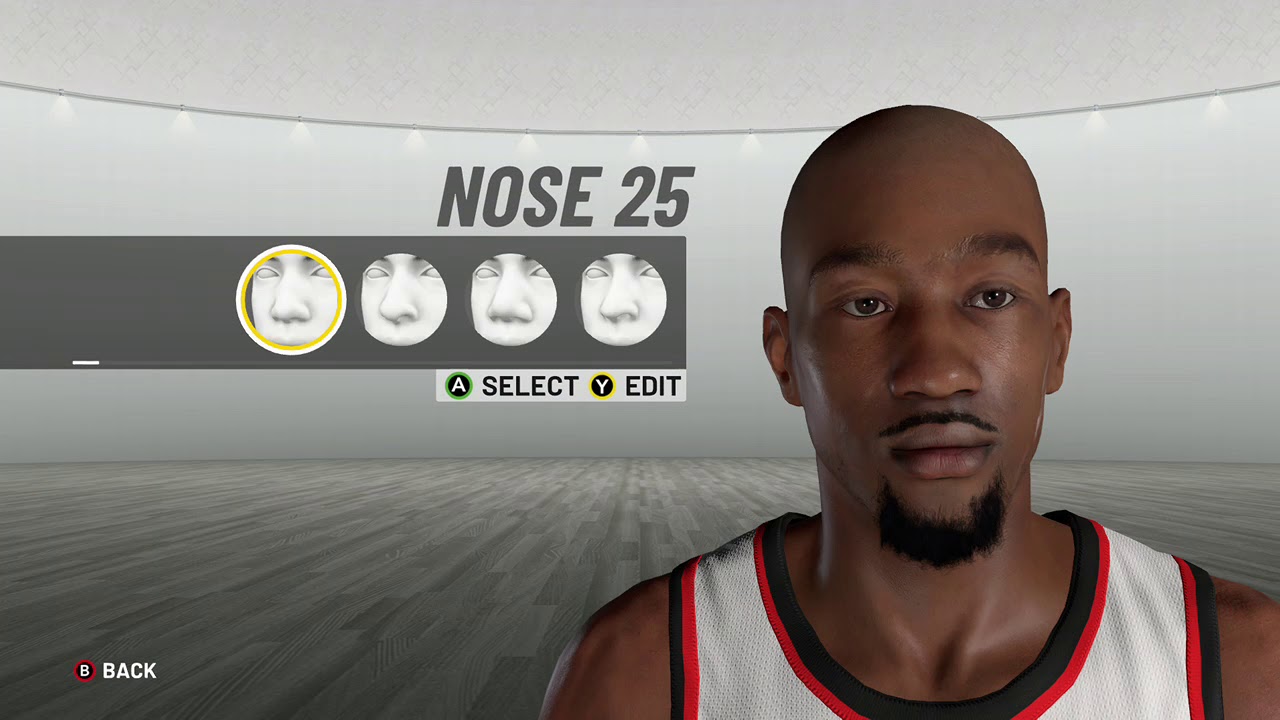This image is a screen capture from what appears to be an NBA 2K video game, showing the character customization screen focused on selecting a nose type. The background features a sleek, modern aesthetic with a grey wood floor and a curved, silver wall. Dominating the center of the screen, the text "Nose 25" is displayed in grey font. 

On the left side, there are four sections featuring different nose options, all displayed on a white 3D model. The selected nose type is highlighted with a yellow ring. Below these selections, the interface shows an "A" button icon labeled "Select" and a "Y" button icon labeled "Edit." 

To the right, a character model is partially visible from the chest upwards. This character sports a bald head, a goatee, and a mustache, and is dressed in a red, white, and black basketball jersey. In the bottom left corner of the screen, an icon of the "B" button is shown with the label "Back." The overall scene emphasizes the customization features available for player avatars in the game.